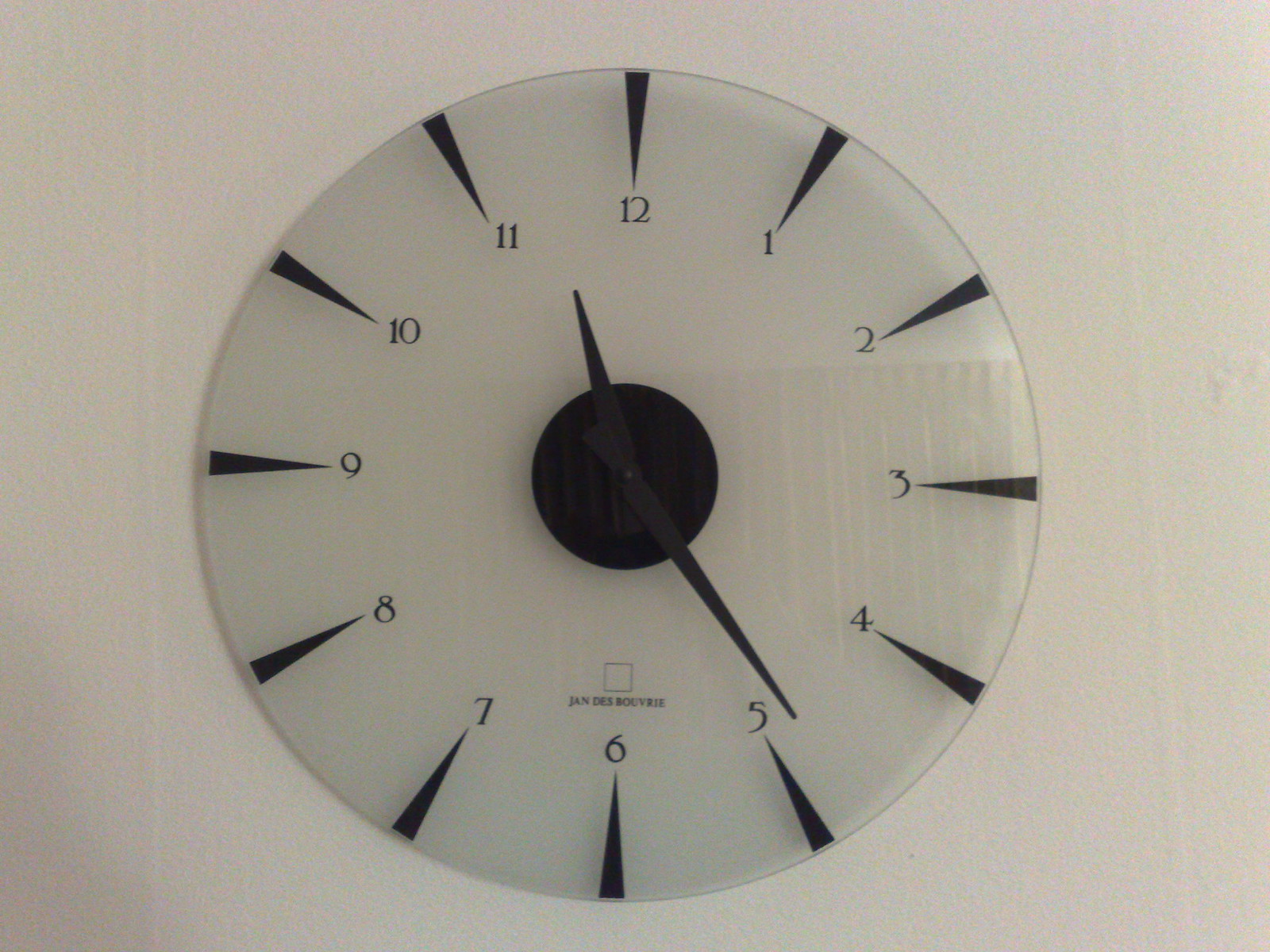This photograph showcases a uniquely designed clock hanging on a wall. The clock is crafted from a piece of thick, yet somewhat transparent, glass resembling a glass plate. Its most striking feature is its minimalistic yet intriguing design. Each hour is marked by a sleek black line that points towards the center, forming a triangle-like shape. There are no minute markers present on the clock face, emphasizing its simplistic aesthetic. A black circle at the center anchors the clock hands – a bold minute hand and a shorter hour hand. The clock shows a time close to 11:24, with the minute hand positioned just before the five and the hour hand slightly past the 11. Additionally, a faint logo or brand mark is visible above the six, though it remains indistinct from the current angle of the photograph. This blend of modern, minimal design with the transparent glass construction makes the clock a captivating, albeit unconventional, timepiece.